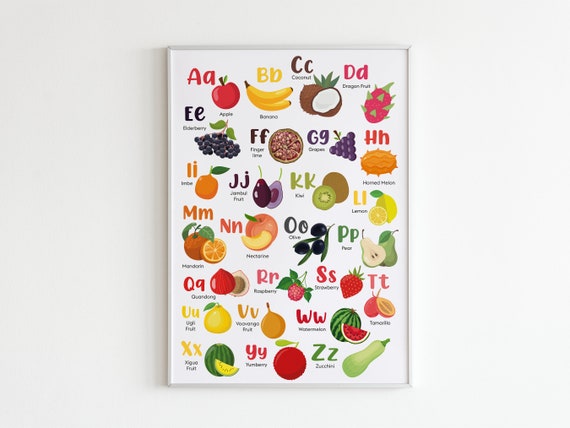The image features a decorative white-framed poster set against a light gray background, showcasing an A to Z guide of fruits and vegetables. The poster is arranged in approximately six rough rows, each corresponding to a letter of the alphabet in a double format—an uppercase and a lowercase letter—paired with an image and the name of the item beneath it in black text. For instance, the top row starts with "A" and "a" in red, alongside a red apple labeled "apple." Next is "B" and "b" in yellow, featuring a yellow banana labeled "banana." This sequence continues, including items like coconuts (brown and white, labeled "coconut") and a spiky dragon fruit. Although some letters and images are difficult to decipher, the poster likely ends with "Z" and "z" for zucchini, while other familiar entries such as strawberries, grapes, and watermelon are included as well.